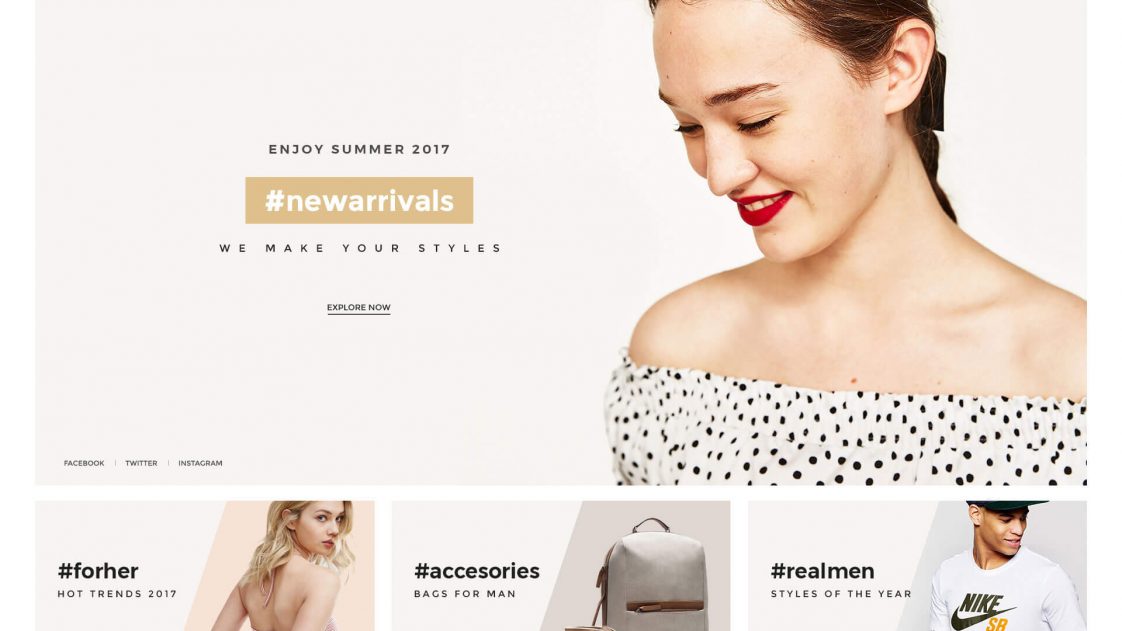**Top Section:**
The image, sourced from a website, features a large banner stretching across the top with a beige background. Centrally, a woman with her brown hair pulled back is showcased. She is adorned with red lipstick and is dressed in an off-the-shoulder beige dress dotted with black polka dots. To her left, bold text reads: "Enjoy Summer 2017 #newarrivals – We make your styles." Beneath this, in smaller print and underlined in black, the invitation "Explore Now" is visible. In the bottom corner of this segment, icons and text for social media platforms—Facebook, Twitter, and Instagram—are displayed.

**Bottom Section:**
Further down, another section emerges featuring different promotional content. On the left, bold text announces "#forher – Hot Trends 2017." Adjacent to this text is an image of a blonde woman wearing a low-back cut shirt. To the right of her, additional text reads "#accessories – Bags for Men," accompanied by an image of a beige bag. The final segment highlights "#realmensstyles of the year," depicting a man clad in a Nike shirt.